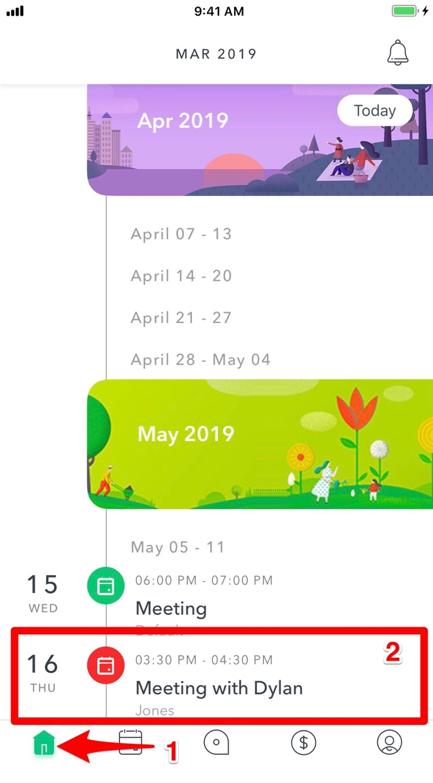This image is a screenshot from an unidentified mobile device, possibly an Android or iOS, given the lack of specific indicators. The background is predominantly white. In the upper right-hand corner, there is a fully charged battery indicator, accompanied by a lightning symbol, signifying that the device is currently charging. The time displayed is 9:41 AM, and the date is March 2019, which is clearly indicated below the time.

The screenshot appears to be from a calendar application, though the layout deviates from a conventional calendar grid. Instead, the days are listed sequentially, one below the next. Each month is introduced with an illustrative image at its beginning. For instance, at the top of the image, April 2019 is marked by an illustration depicting people having a picnic on a beach. Below this, the weeks of April are displayed: April 7th-13th, April 14th-20th, and April 21st-27th, suggesting that users can click on them for more detailed information.

A notable feature of the screenshot is a highlighted section at the bottom for the date May 16th. This date is emphasized with a red box that includes a specific event: a meeting with Dylan scheduled from 3:30 to 4:30 PM.